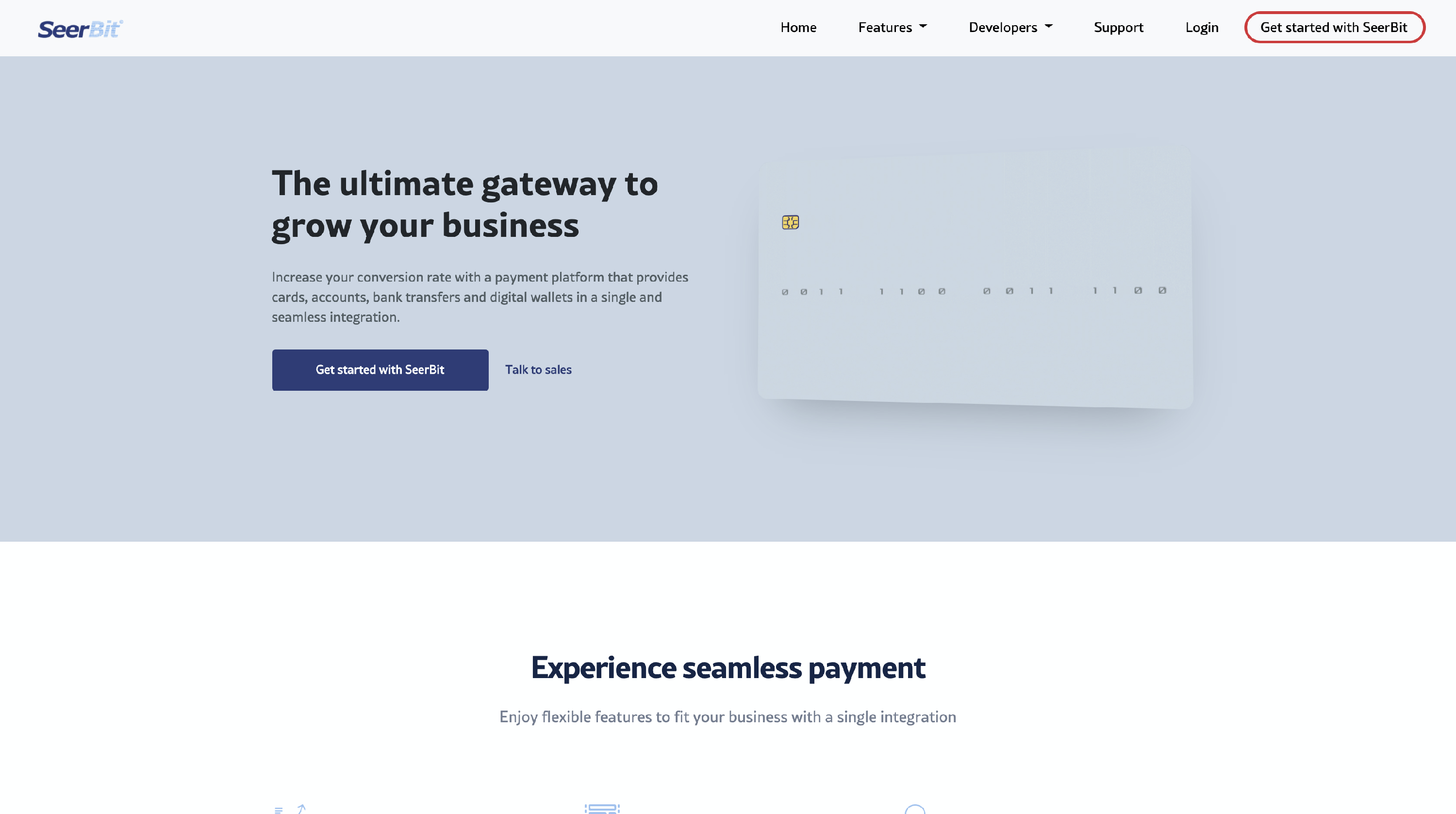This is a detailed screenshot of the SeerBit website. In the upper left-hand corner, the SeerBit logo is prominently displayed in blue. Adjacent to the logo are several menu options arranged horizontally: Home, Features, Developers, Support, Login, and Get Started with SeerBit. The latter stands out with its call-to-action emphasis.

Beneath the navigation bar, a large bluish-gray banner spans the width of the page. In the center of this section, bold black text declares, "The Ultimate Gateway to Grow Your Business." Directly below this statement, a striking blue button invites users to "Get Started with SeerBit."

Further down, additional black text reads, "Experience Seamless Payment, Enjoy Flexible Features to Fit Your Business with a Single Integration," further emphasizing the service's streamlined and adaptable payment processing capabilities. This suggests that SeerBit is a payment receiving and sending service designed to simplify financial transactions for businesses.